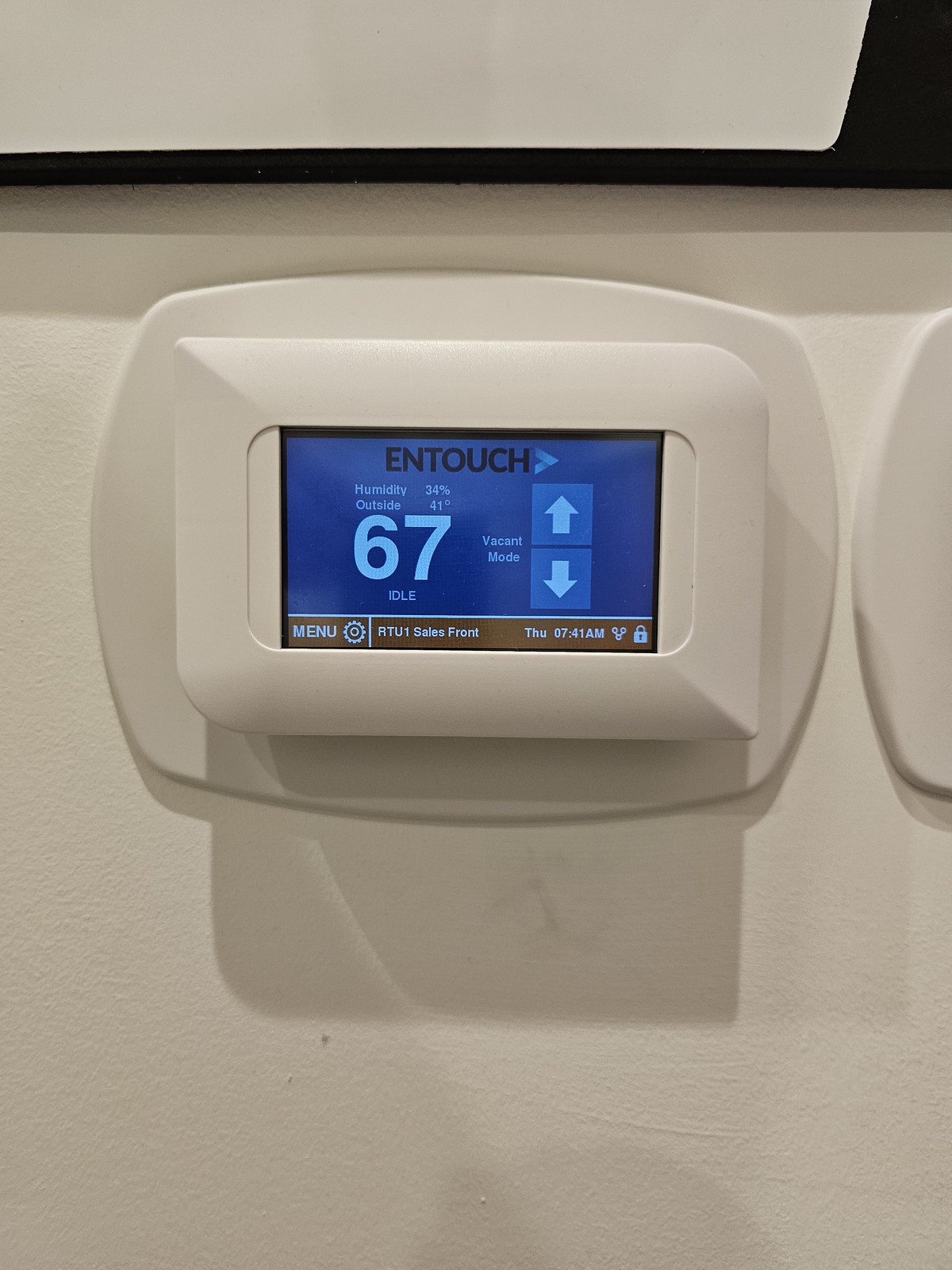The photograph shows a small digital screen display set within a horizontal rectangular frame made of white plastic. The frame is distinctive with unique pointed corners on the upper left and lower right, and rounded corners on the lower left and upper right. This frame protrudes slightly from a slightly larger white panel behind it. To the right, only the edge of a second, identical panel is visible before the image cuts off, suggesting a series of similar displays.

These panels are mounted on a pristine white wall. Just above them, a thin black strip runs horizontally across the image, making an L-shape as it extends vertically to the upper right corner. The upper and left sections of the image are predominantly white.

Focusing on the digital display, the screen is primarily blue with a thin brown strip along the bottom. This strip features a 'Menu' button on the left, the current date and time, and various settings icons on the right. The large blue section of the screen prominently displays the number '67' in white on the left, likely indicating the indoor temperature. Above this number are small readings, possibly for humidity and outside temperature, though the font is too small to be legible.

The right half of the screen includes square buttons with white up and down arrows for adjusting settings. Across the top of the screen, in black uppercase letters, it reads "READS" and "TOUCH."